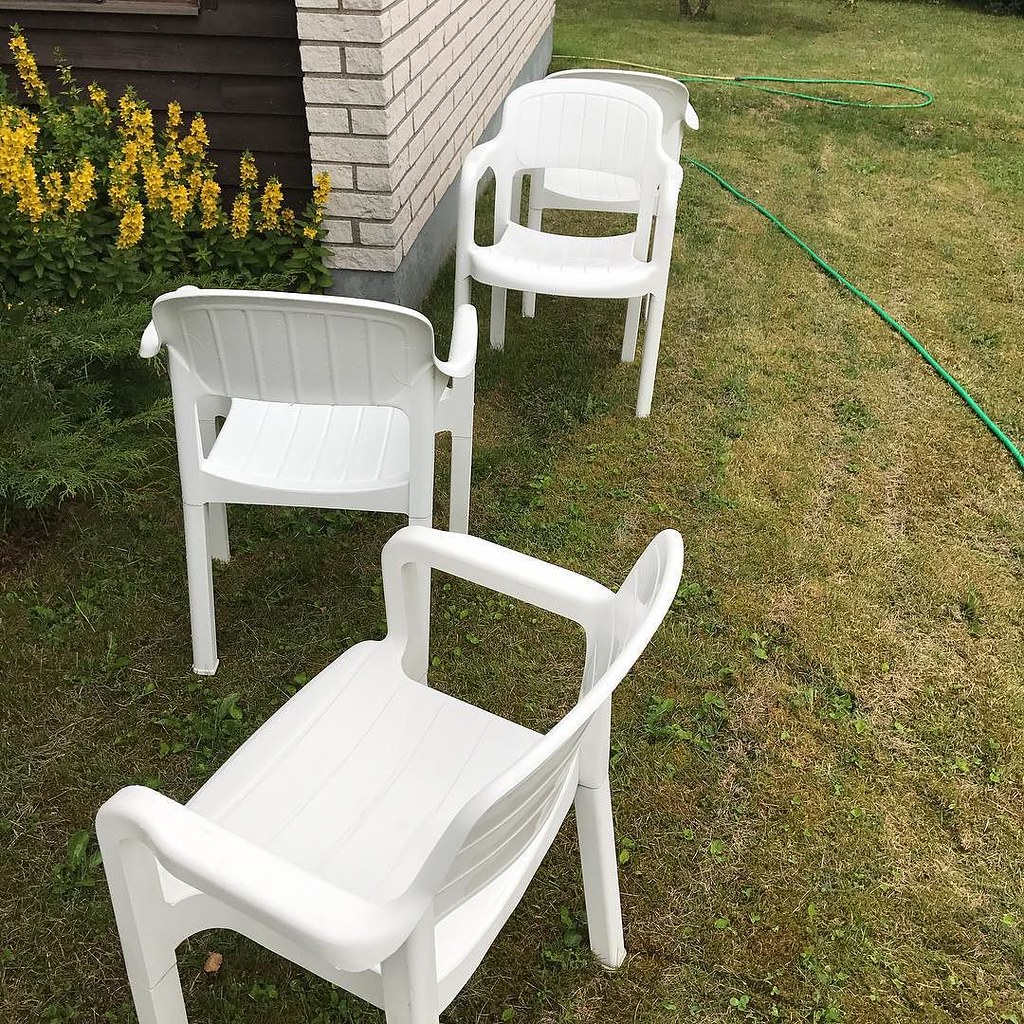This outdoor image is marked by a combination of natural and man-made elements. Dominating the left side is a white brick structure with a gray bottom; attached to it is a section of dark brown wood. In front of this structure stands a lush green bush adorned with yellow flowers, which extend upward like a ladder. The ground is covered in well-manicured grass. Scattered across the lawn, four identical white plastic chairs are arranged in a somewhat haphazard fashion, with their backs turned to one another. Two of these chairs are located directly to the right of the building, both facing different directions. Below the brick structure, the remaining chairs are positioned diagonally and vertically. A green water hose snakes its way from the right side of the photograph, trailing across the grass and heading behind the brick building. The combination of the horticultural elements, the arrangement of the chairs, and the presence of the hose create an intricate outdoor setting.